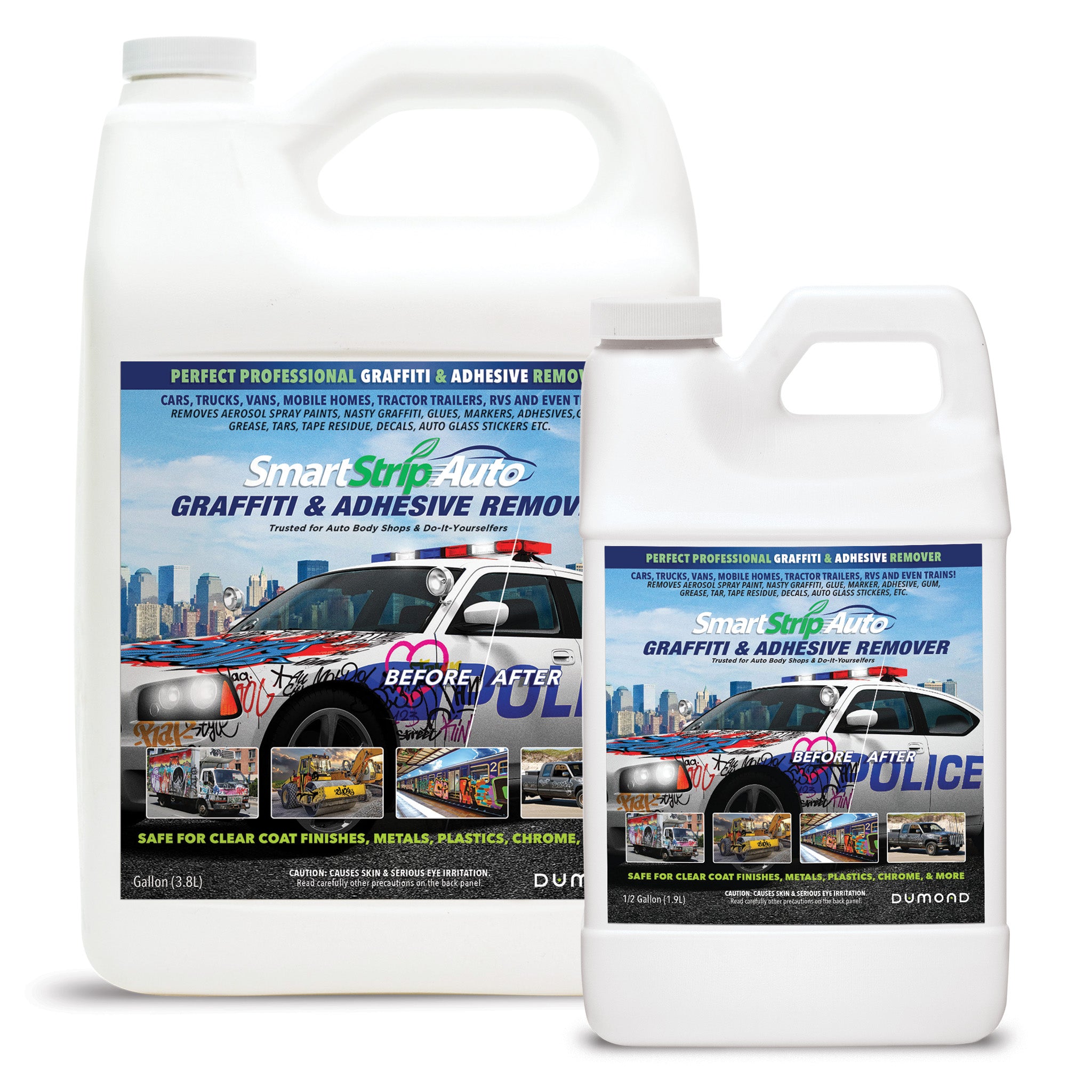In this image, set against a stark white background, we see two large plastic containers—one large and one smaller—both similar in shape to those commonly used for holding antifreeze. Each container is all-white and features a detailed label. The prominent label on the larger container prominently displays a blue background with a detailed city skyline and a police car in the foreground. The police car is noticeably covered in graffiti. The label reads "Perfect Professional Graffiti and Adhesive Remover," followed by "Smart Strip Auto Graffiti and Adhesive Remover." Beneath the image of the police car, there are additional smaller images depicting various scenarios: a graffiti-covered truck, heavy machinery marked with graffiti, the side of a subway train with graffiti, and finally, a gray pickup truck defaced with graffiti. These images illustrate the product's versatility and effectiveness in removing graffiti from different types of vehicles and surfaces.